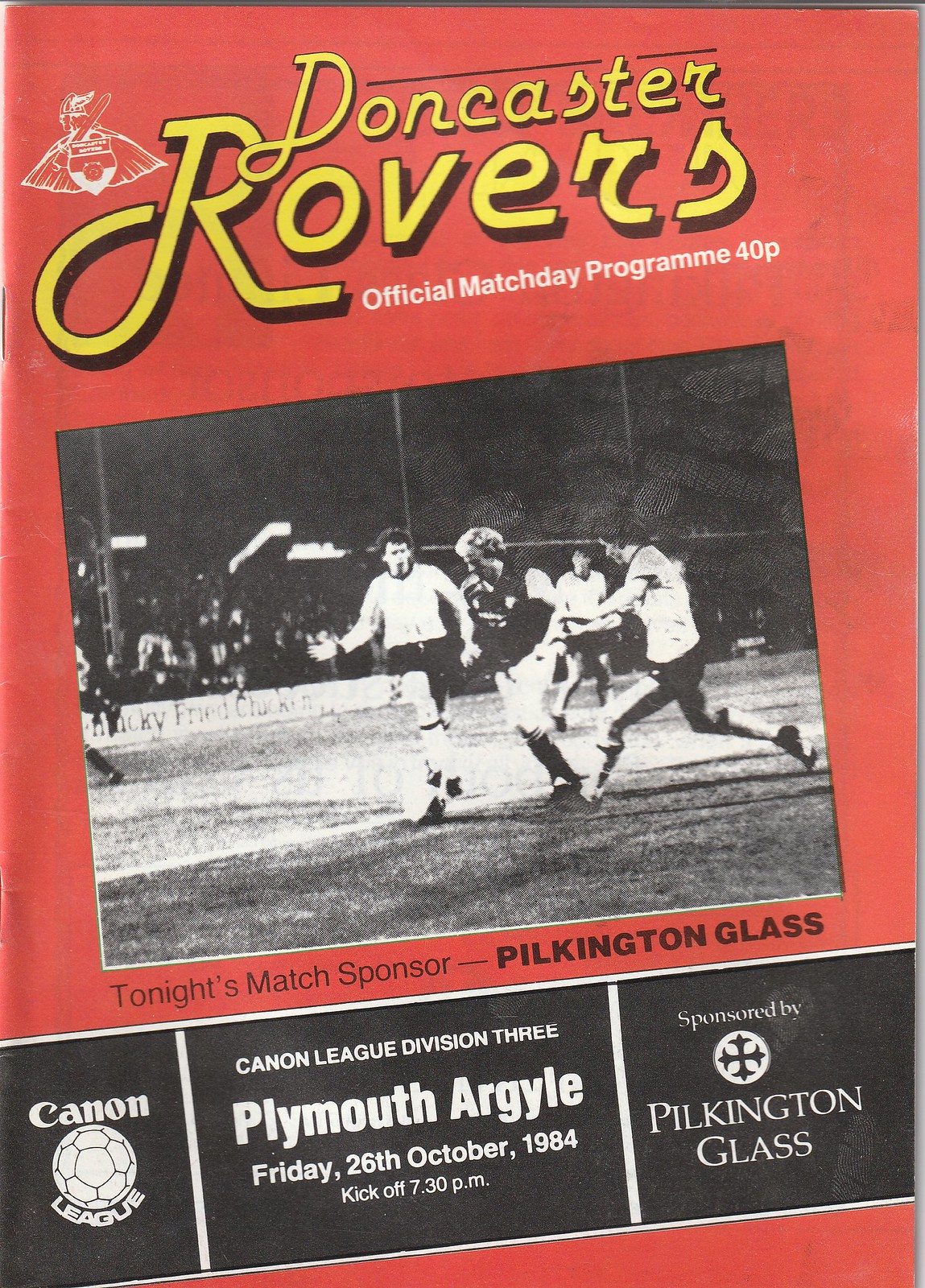The image is the front cover of an official match day program for the Doncaster Rovers, priced at 40 pence. The cover features a bold, yellow graphic font at the top that reads "Doncaster Rovers," accompanied by an insignia in white. In the center, there is a prominent black and white photograph of several football players in action on a field, with fans faintly visible in the background. Below the image, the text details "Tonight's Match: Pilkington Glass," and states that the game is part of the Canon League Division 3 against Plymouth Argyle, scheduled for Friday, 26th October 1984, with kickoff at 7:30 p.m. The cover also includes the logos of Pilkington Glass, emphasizing their role as the match sponsor, along with various other advertisements. The overall design uses a color scheme of red, white, yellow, gray, black, and brown, and the placement of elements is structured with the team name at the top and the sponsors at the bottom, reflecting the official and organized nature of a program typically distributed at soccer matches.